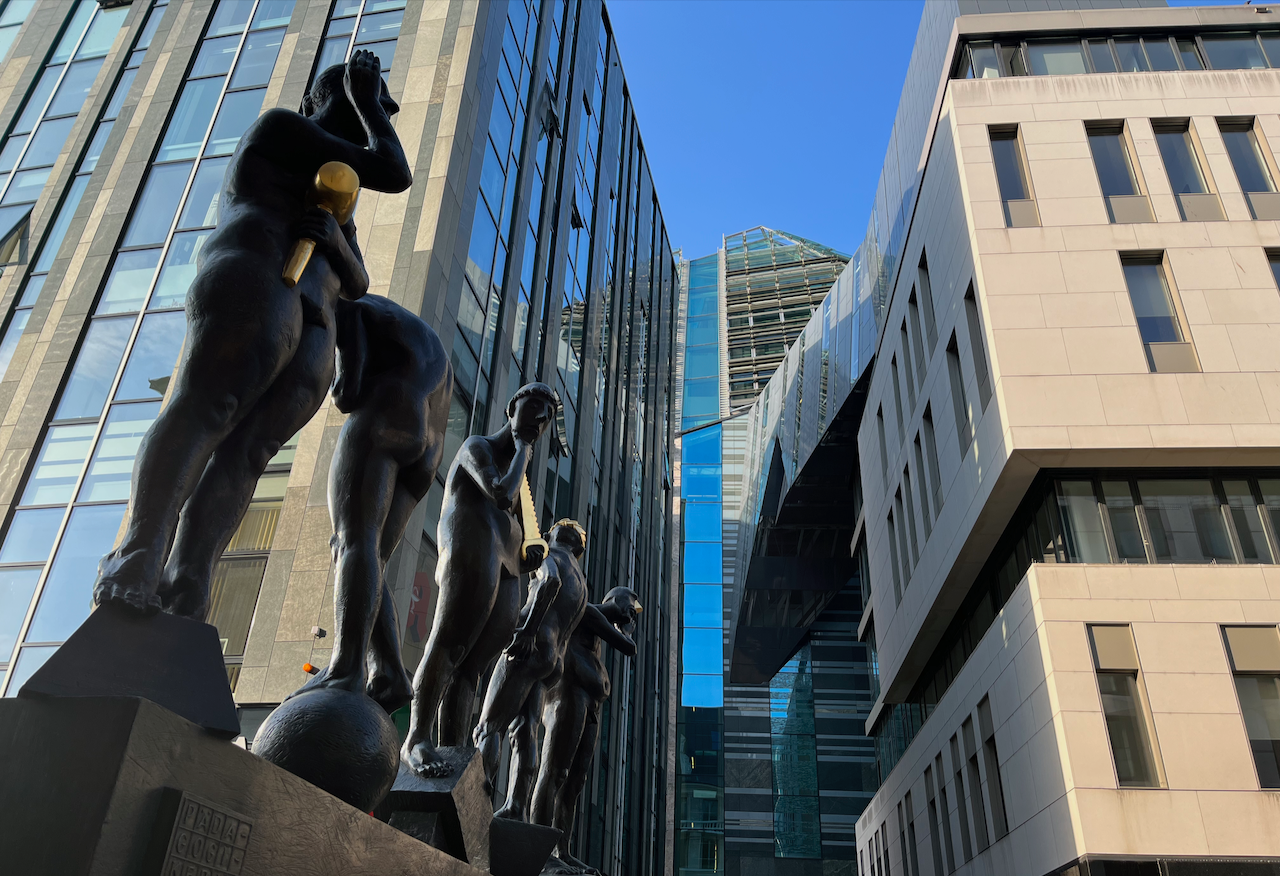This landscape-oriented photograph captures a striking series of statues set against an urban backdrop of modern skyscrapers. Positioned slightly to the left of center and arranged in a line, these dark metal statues depict naked human figures in various poses and bodily shapes, each standing on unique geometric pedestals such as a trapezoid, sphere, and cube. The figures are slightly abstract, possibly half-human and half-animal, and they alternate in their orientation, facing either left or right. 

The frontmost statue is a person facing right, holding a golden mallet under a raised arm. Behind it, a figure faces left partially obscured, while the third statue, a man with a bowl cut and beard, faces right and clutches a golden saw. The fourth figure, hidden and facing left, remains partially out of view. The final statue, a pot-bellied man, holds an undiscernible item close to his ear. 

Surrounding the statues, the urban environment boasts modern architecture. A sleek glass skyscraper with vertical columns occupies the left side, while straight ahead another glass building features a column of windows rising up to an angled top resembling a pyramid. To the right, a brownish building with rectangular glass windows completes this vivid tableau. Above, a sliver of blue sky adds a touch of color to the scene.